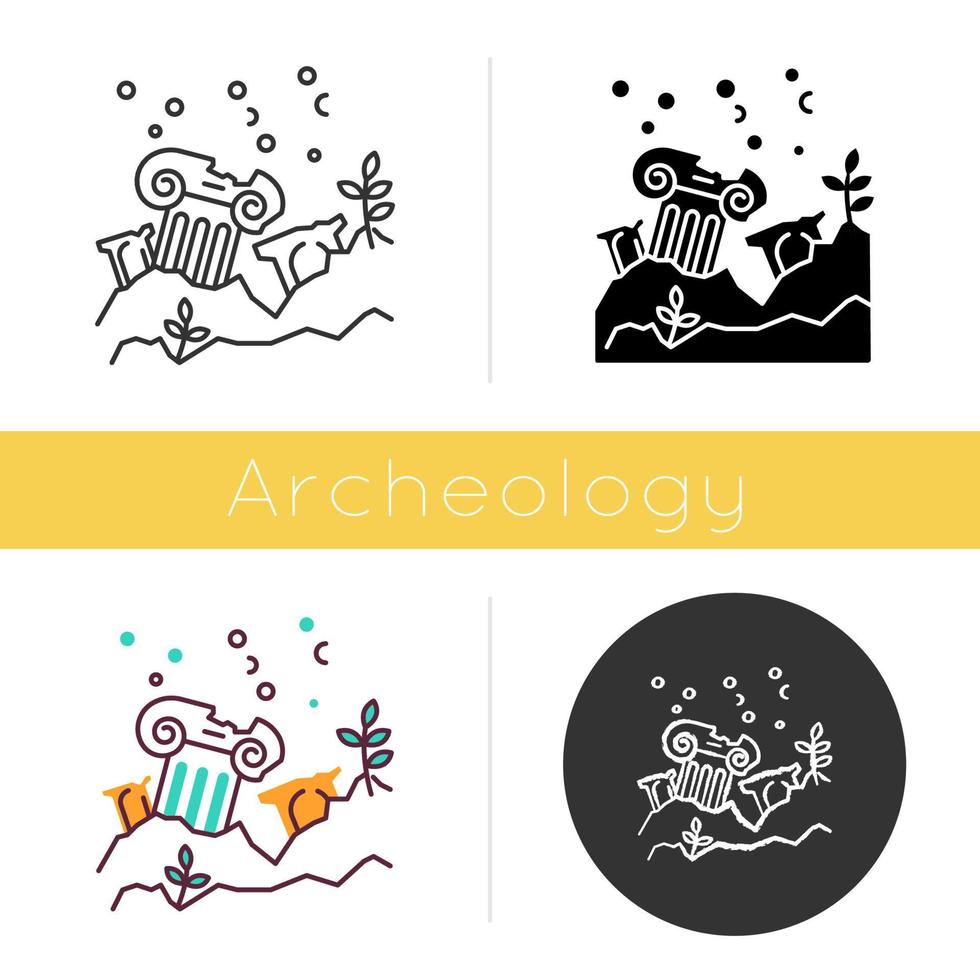The image is divided into four quadrants, each featuring a repeated illustration but with different color schemes and styles. Central to the image is a pale orange-yellow horizontal bar that prominently displays the word “ARCHAEOLOGY” in white text. In the top left quadrant, we see a black line illustration on a white background depicting a cartoony scene of crumbling columns and a rocky area with small plants and bubbles. The top right quadrant showcases a negative version of the same image, where the black outlines are filled in, making it appear as an inverted black-and-white design. The bottom left quadrant displays the same scene, but this time in color: the bubbles are light teal, while the pillars feature gold and light blue hues. Finally, the bottom right quadrant shows the image again, this time in white on a fully black background with the entire composition enclosed in a black circle. The detailed variations in color and style across the four images all revolve around the central archaeology theme.